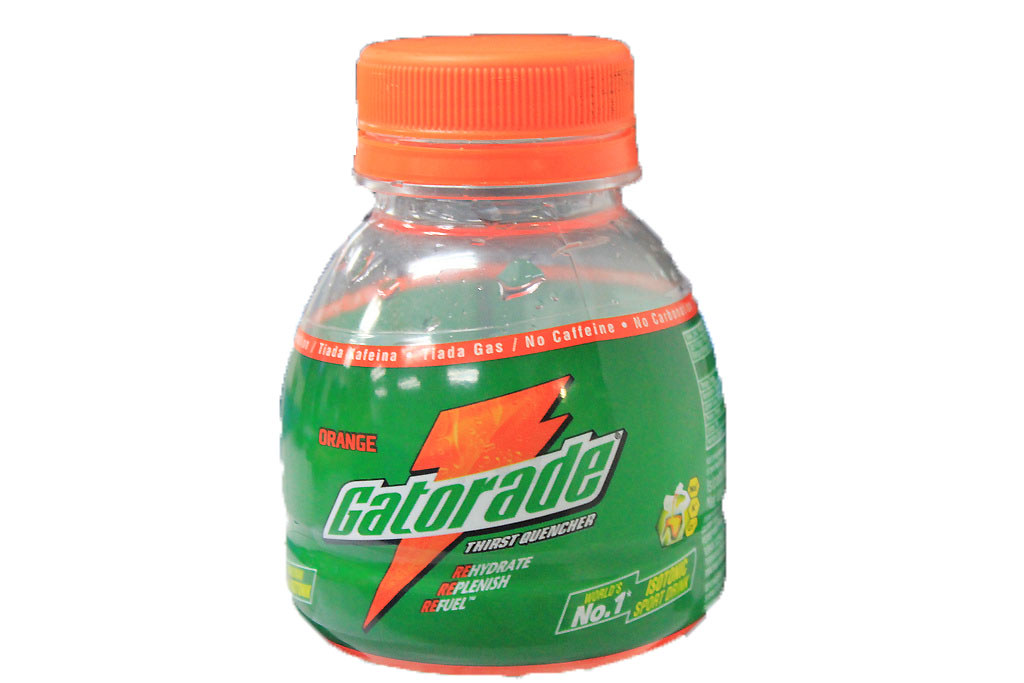The image features a distinctive, compact bottle with a vibrant design. The bottle is topped with an orange cap adorned with ridges for grip. Below the cap, there is a transparent section followed by another orange ring. The middle section of the bottle is made of clear plastic, showcasing the liquid inside. Encircling the bottle is a bold orange stripe, emblazoned with text that reads "Gatorade, Thirst Quencher, Rehydrate, Quench, Refill." Centrally placed on the bottle is a prominent green label, adding to the visual appeal. In the top right corner of the bottle, there is an indication that it ranks as the "#1" in something, possibly hinting at its popularity or leading status.